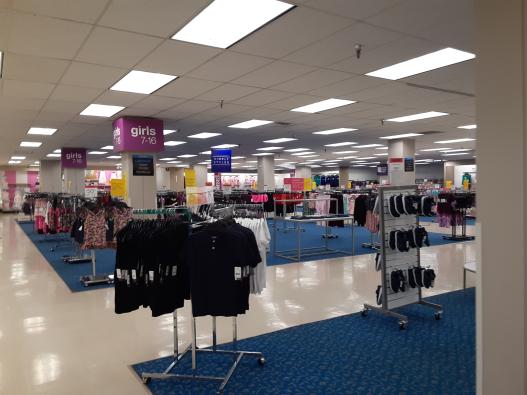The photograph captures the interior of a large, well-lit department store, likely reminiscent of a Target or Walmart. The image reveals a spacious floor layout filled with various clothing racks and displays. The clothing section prominently displays items for girls aged 7 to 16, as indicated by a labeled sign in purple on a support pillar. The floor combines blue carpeting with white linoleum walkways, enhancing the organized retail space. On the upper part of the image, the ceiling is covered with cardboard tiles interspersed with rows of fluorescent sheet lighting, ensuring the entire area is brightly illuminated. The racks are adorned with a variety of items, including t-shirts, sandals, tops, and flip-flops. The photo appears to be taken from near the entrance, providing a wide-angle view that encompasses much of the store's layout, inviting viewers to explore the detailed and highly organized clothing section.